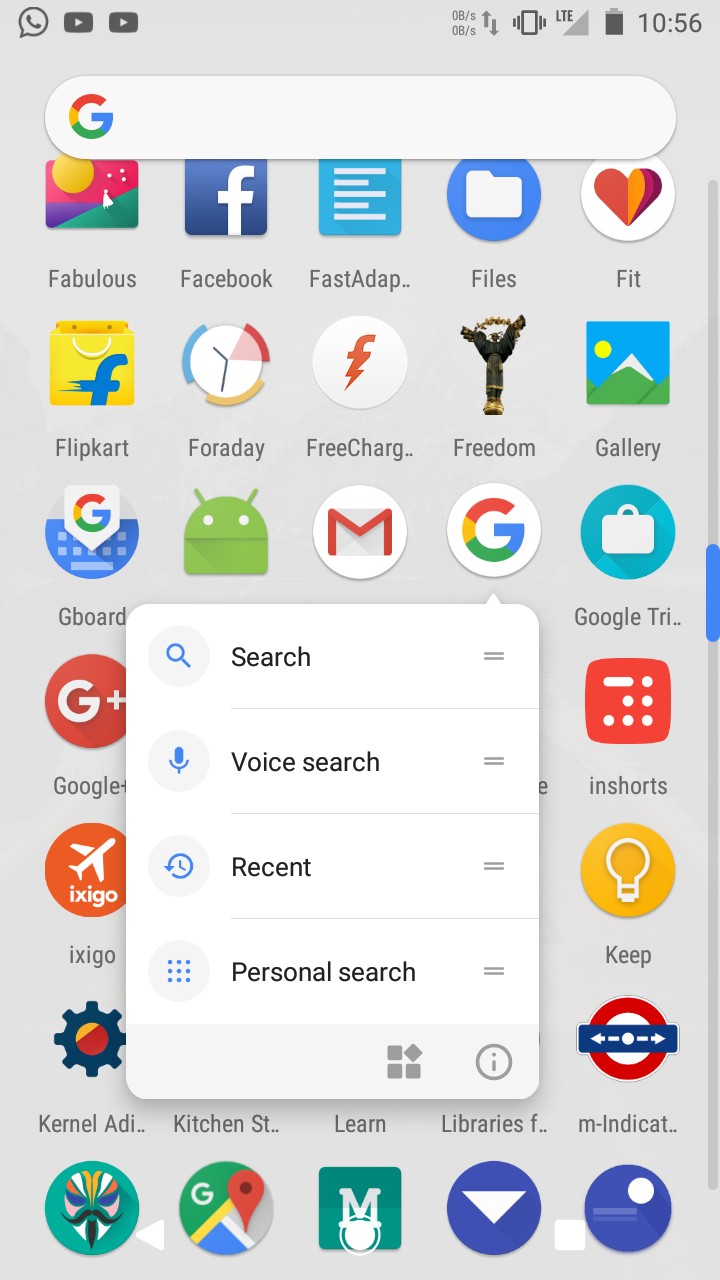The image depicts a smartphone screen displaying the main app menu. In the upper-left corner, there is a phone icon, indicating the dialer app. Adjacent to it, there are two YouTube icons, recognizable by their black boxes with white play arrows pointing to the right. The status bar at the top of the screen shows icons representing signal strength, battery life, and the current time.

Beneath the status bar is a white, oblong search box adorned with the colorful Google logo, emphasizing that it is a Google search bar. The background of the screen is gray, and the app menu is organized into a grid of seven rows and five columns, with each icon representing a different app. The apps appear to be arranged alphabetically, as indicated by the labels beneath each icon.

Overlaying this app grid is a white pop-up box offering search functionalities, including a standard search, voice search, and recent personal searches, suggesting a feature that allows users to easily locate specific apps or perform quick online searches.